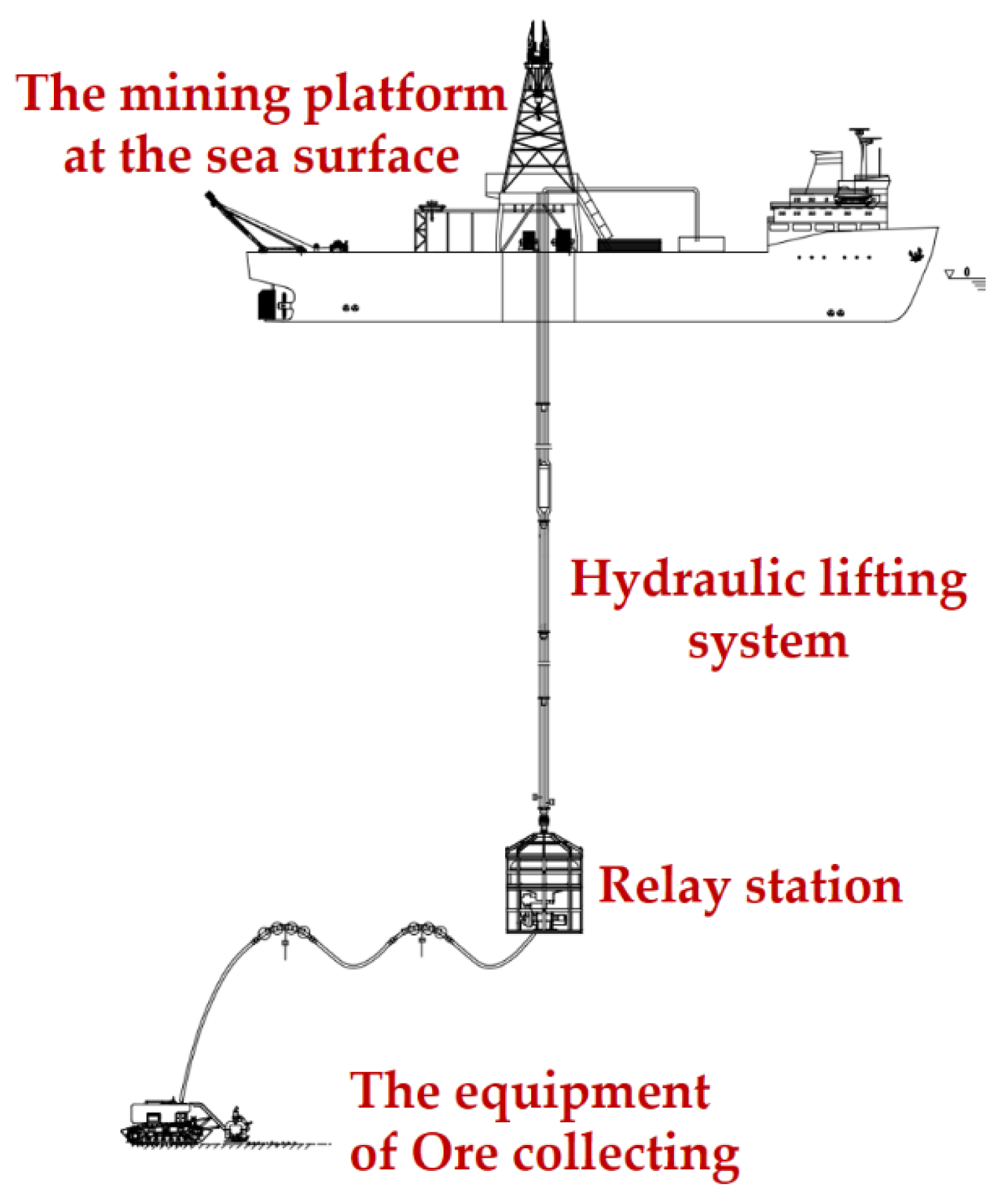This detailed diagram illustrates a black-and-white, 2D-rendered ship representing a mining platform at the sea surface, with key elements highlighted in red text. From the ship, a pipe descends vertically into the water, labeled as the "hydraulic lifting system." At the bottom of this pipe lies a "relay station," also marked in red. Extending from the relay station, another line reaches a piece of heavy machinery identified as the "equipment of ore collecting." The entire setup suggests a complex underwater mining operation, possibly depicted for educational or instructional purposes. The red text annotations guide the viewer through the sequence, from the mining platform at the surface to the ore collection apparatus on the sea floor.